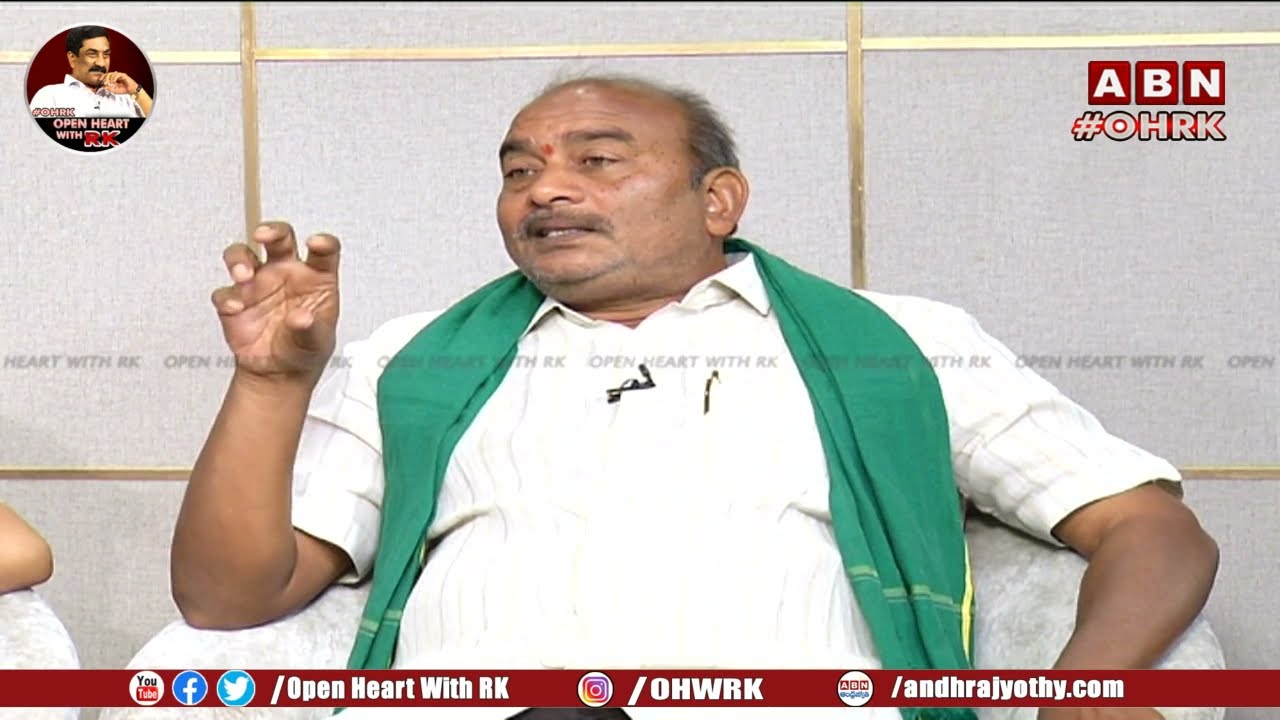This image depicts a serious-looking older Indian man, possibly being interviewed on a television program. He sits with a white collared shirt and a green towel draped across his shoulders. His right arm is bent at the elbow, with his hand open as if demonstrating something. He sports a bit of a mustache and a day-old stubble beard. Notably, he has a red dot in the middle of his forehead, light-colored eyes, and grayish dark hair; he is also partially bald and has very thick eyebrows. There is a red banner at the bottom of the screen featuring logos for YouTube, Facebook, Twitter, and Instagram, accompanied by text that reads 'Open Heart with R.K.' and 'OndraJayothi.com'. The upper part of the screen includes various text elements: the upper left has a watermark with an image of a man and the text 'Open Heart with R.K.', while the upper right displays 'A.B.N. #O.H.R.K.' Behind the man is a gray dividing panel, and there is a glimpse of another individual’s elbow and chair in the bottom right corner.